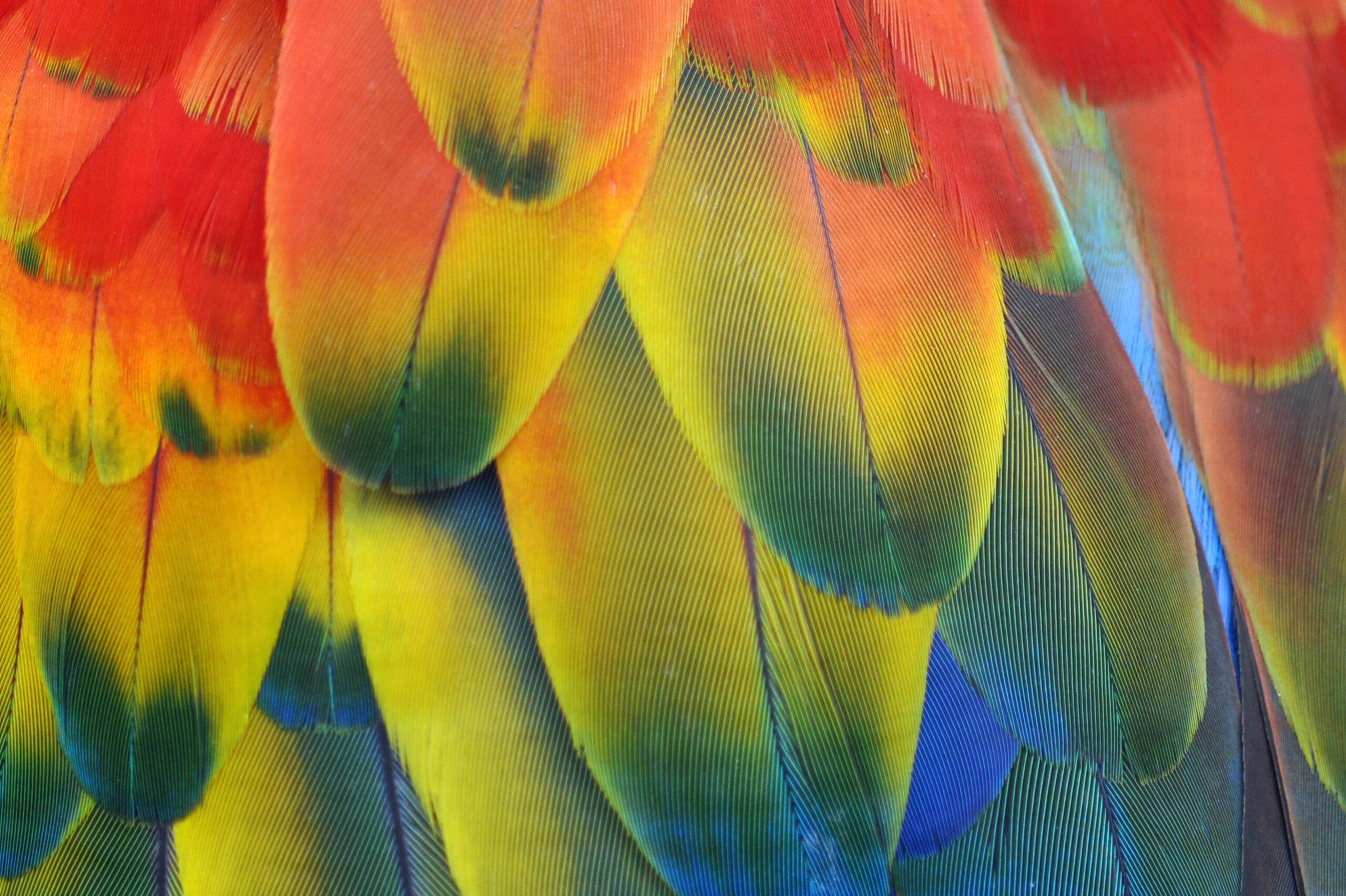The image depicts an intricate design featuring an array of vertically hanging, oval-shaped objects. The top portions of these objects are predominantly red, with some displaying light pink patches. The lower sections transition to yellow, accented with dark green patches at the tips. Towards the right-hand side, a few objects exhibit a gradient from purple to green, concluding with yellow hues. In the center, the objects start as yellow and gradually shift to blue. The left side repeats this yellow-to-blue gradient, while the right-hand side predominantly showcases a blend of blue and purple shades.